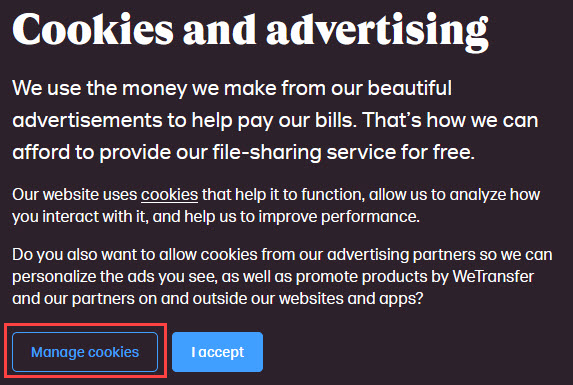**Detailed Caption:**

This is a screenshot from a file-sharing application, showcasing an important disclaimer about their advertising and cookie policy. The image features a stark black background with predominantly white text, making the message highly visible and easy to read. At the top of the image, enlarged white font prominently displays the words "Cookies and Advertising." The content clearly communicates that the file-sharing service funds its operations through advertisements, which allows them to offer their services to users free of charge.

Further down, the text elaborates: "We use the money we make from our beautiful advertisements to help pay our bills. That's how we can afford to provide our file-sharing service for free." This statement transparently informs users about the financial model behind the free service.

Additionally, the disclaimer advises users about the role of cookies in this process, explaining that by allowing cookies to track their browsing sessions, users contribute to the service's revenue stream. At the bottom of the image, there are two actionable buttons for users to choose from: "Manage Cookies" and "I Accept." The "I Accept" button is blue with white text, signifying an easy acceptance of the policy. The "Manage Cookies" button, which is black with blue text and highlighted with a red box, directs users toward customizing their cookie preferences.

The red box around the "Manage Cookies" button emphasizes that the image serves as instructions on setting cookie preferences, guiding the reader on how to exercise control over their privacy settings. This vivid and concise layout ensures users understand the implications of their choice, providing a clear and striking visual message on a dark background with bright white text.